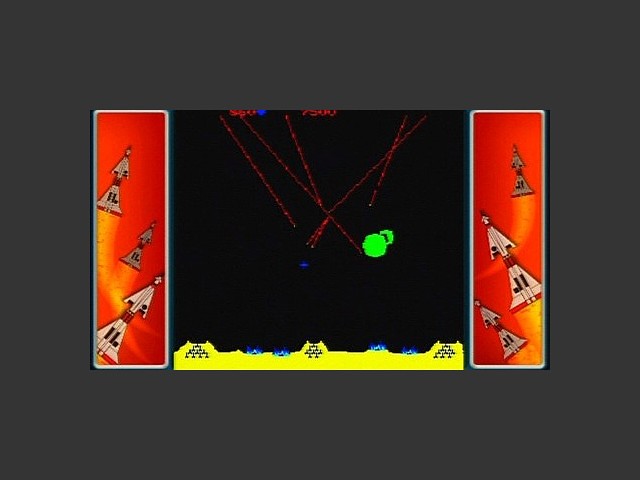In this image, we observe a screen capture from a video game. The backdrop features a grey color scheme, framing the game screen at the center. On either side of the central game display, there are two tall red rectangles adorned with rocket ship graphics, from which yellow flames are prominently visible. At the bottom of the game screen, there's a band of yellow, possibly representing a ground or base layer. Above that, the gameplay area is displayed. Within this area, towards the right, there are two noticeable green dots, while more towards the center-left, a small blue light can be seen. Additionally, striking red lasers are projecting downwards from the top of the screen, adding a dynamic and intense visual element to the scene.